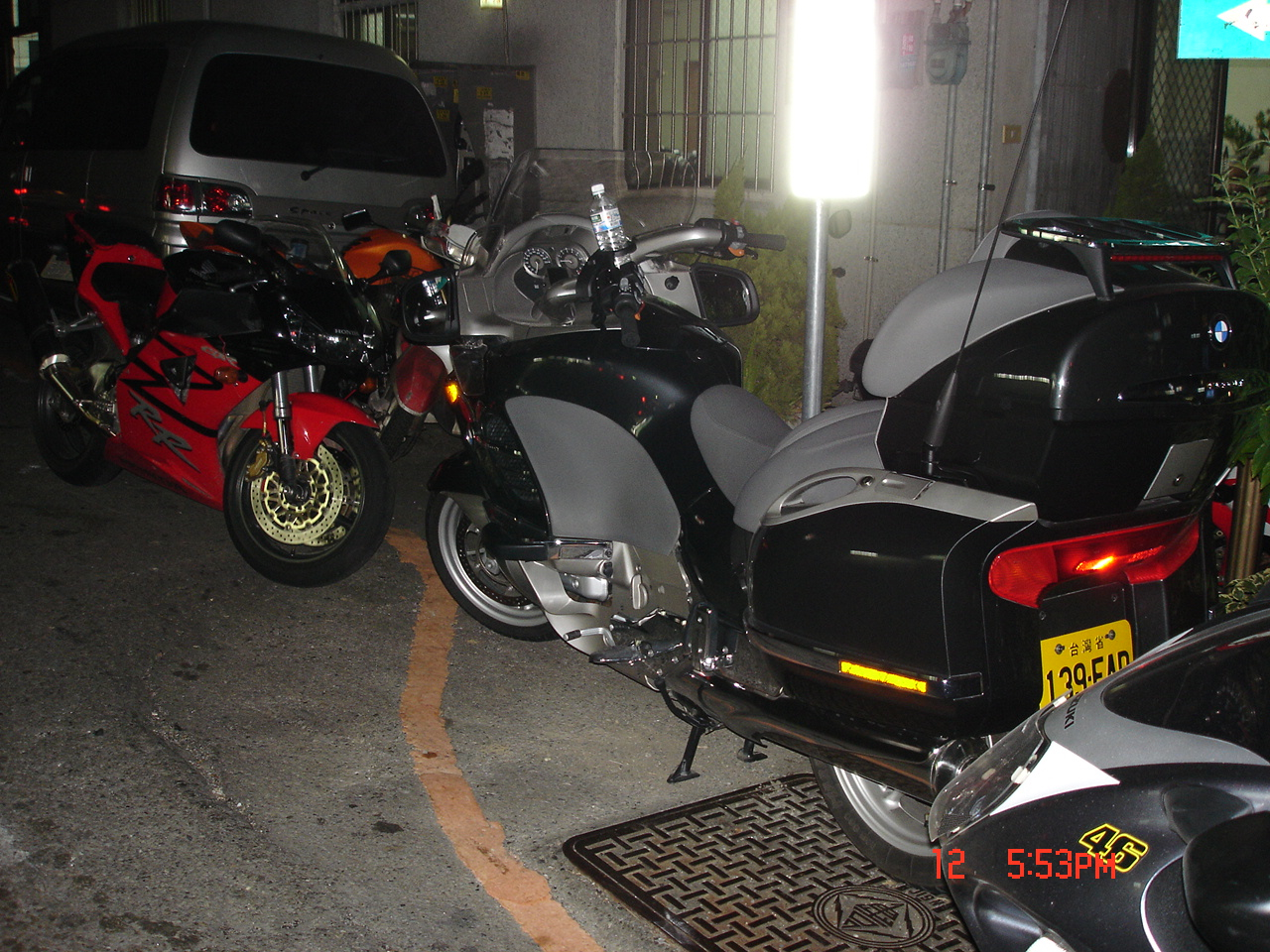This nighttime photograph, taken with flash, captures a bustling street scene that appears to be outside a house or pub. Positioned behind a red and yellow road stripe indicating a parking area, the image prominently features multiple motorbikes and a large silver van with black tinted windows. The centerpiece is a black and silver motorcycle with substantial side saddles, potentially a Harley Davidson, sporting a yellow number plate that starts with "139". A bright red motorbike and a large scooter-like vehicle share the space, with one bike's back wheel parked over a drain grid. Close by, two smaller sports bikes labeled "RR" and a possibly Suzuki-branded unit are visible, highlighting the variety of vehicles. The silver van, partly obscured, displays the number "46" outlined in yellow. The backdrop reveals a white building adorned with burglar bars on its windows, a bright light attached to a pole, and a small bush placed between the van and the structure. An unmanageable road sign further attests to the flash's intensity, adding to the scene's vibrant and lively atmosphere.